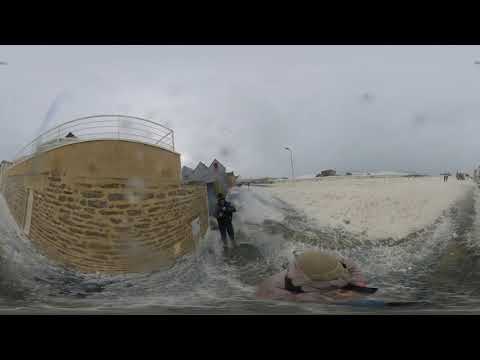The image is a badly out-of-focus, horizontally rectangular color photograph, bordered in black on the top and bottom, taken outdoors in what appears to be inclement weather. Dominating the left side of the image is a curved brown brick structure with a flat top, accentuated by a metal railing. On the far left, there seems to be a door, while the far right features a human figure dressed in black, standing in what looks like water, suggesting a flood or a high-flowing dam. The background reveals a few houses, a distant streetlamp, and a gray overcast sky, further hinting at stormy conditions. Adding to the scene's chaotic ambiance, there are specks of water on the camera, reinforcing the impression of either a snowstorm or flash flood. Overall, the image conveys a sense of urgency and confusion due to the severe weather and the chaotic water flow.